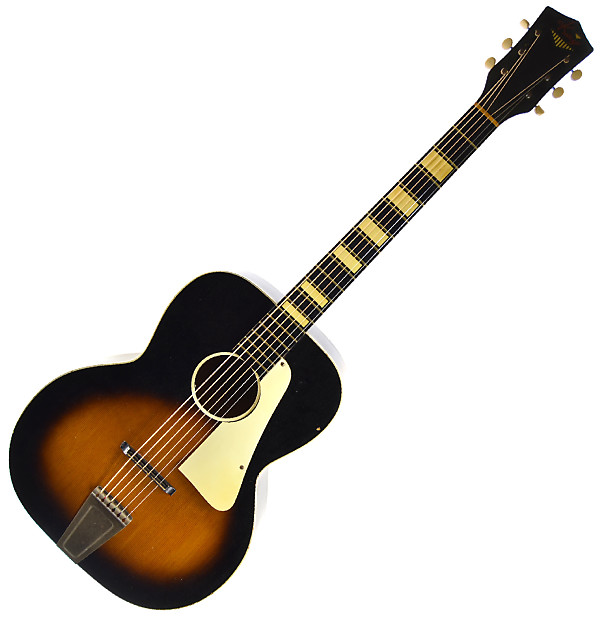This color photograph features a six-string acoustic guitar set against a white background, angled upward to the right. The guitar has a black headstock and fretboard adorned with yellow line segments, and yellow tuning machines at the top. The body of the guitar is black and brown, with a darker black shade around the edges and a lighter brown in the center. It also has a light yellow pickguard on the right side to protect from strumming. The head of the guitar is somewhat rectangular with a slight point, and it includes a section that appears to be white plastic.